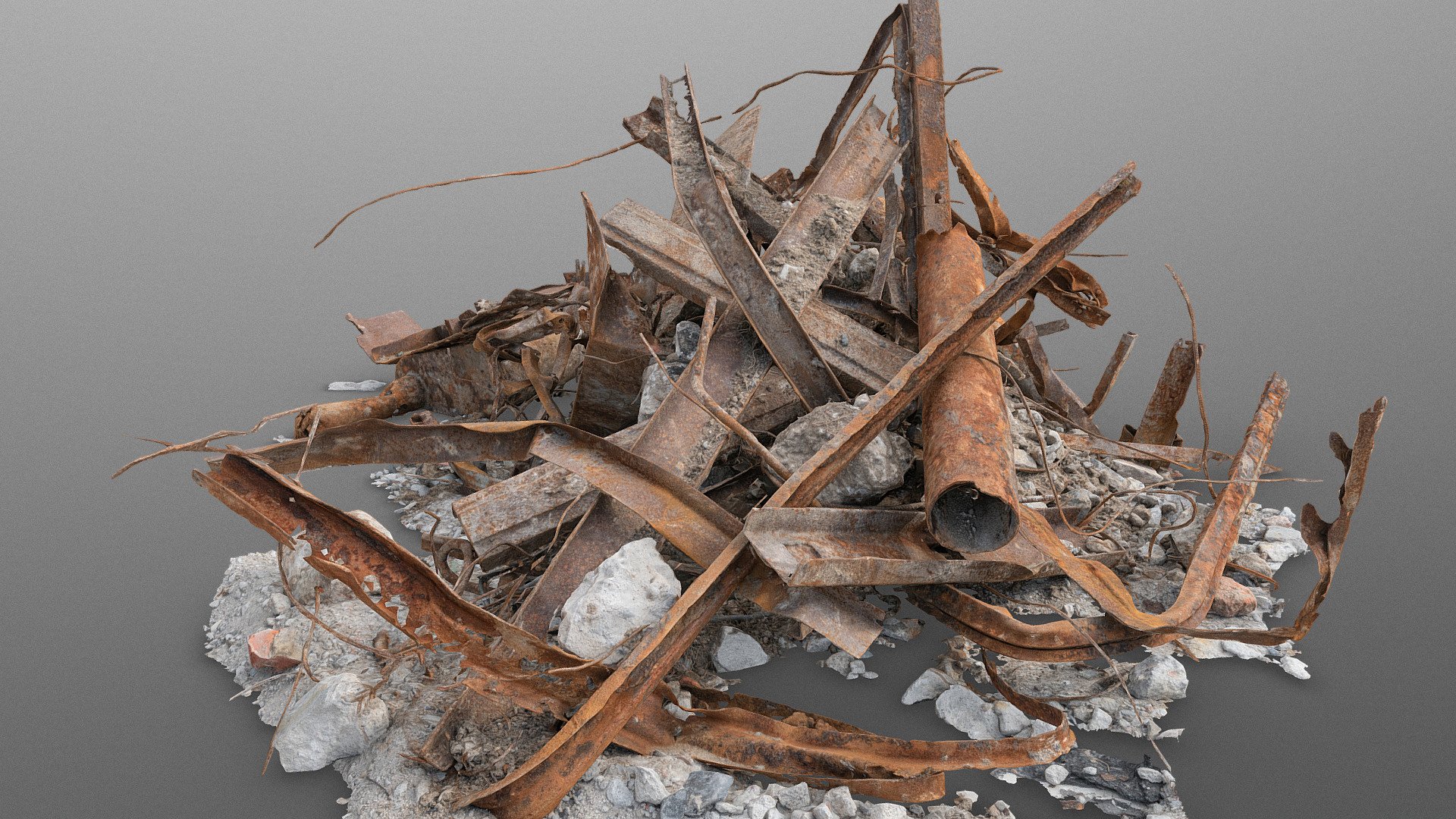This image captures a central pile of rubble against a solid gray background, possibly suggesting a derelict construction site. Dominating the scene are disordered, rusted metal pieces, including long, rectangular beams bent and curled, and a large cylindrical pipe lying horizontally on top. Interspersed amongst the metal are varying sizes of stones and pebbles, ranging from white to darker gray, all dusted with a layer of concrete and gray dirt. Additionally, a tangle of thin, reddish-brown wire snakes through the mass, contributing to the chaotic yet intriguing composition of the debris. The muted gray background, which occupies most of the image, contrasts sharply with the textured and rusty hues of the rubble.